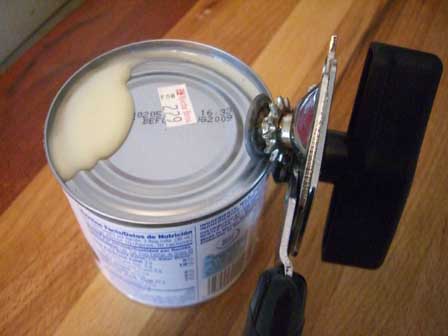This photograph captures the moment a black-handled can opener is methodically slicing into a partially opened aluminum can, revealing a light, white-ish liquid, possibly condensed milk or cream, seeping from the incisions. The can, positioned on a wooden counter, displays a plain white label with blue writing, some nutritional information, and a small red store name printed on a white rectangular sticker showing the price "$2.29." The lid, clamped by the can opener's metallic wheel and black turning knob, features additional black-stamped information, including an expiration date. The can opener itself, partially obscured by the can, shows no human hand, suggesting the captured moment focuses purely on the interaction between the tools and the can.